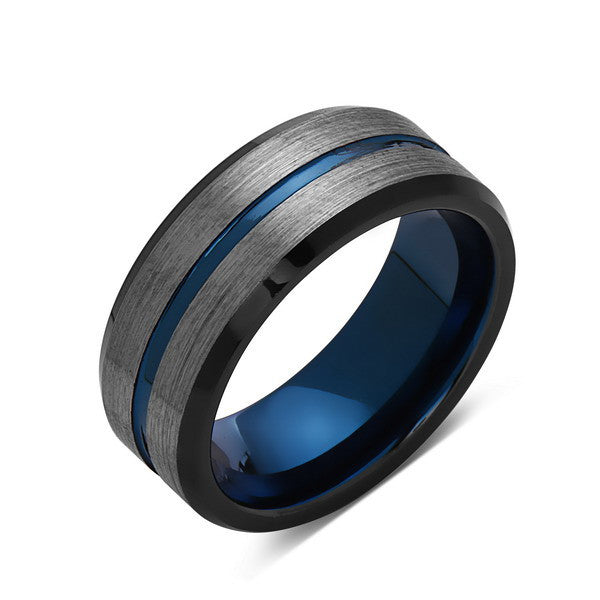This is an ultra-close, detailed image of a sophisticated silicone wedding band, meticulously designed to resemble a traditional metallic ring. The band features a striking royal deep blue stripe running through the center of its sleek, gray exterior, which mimics the appearance of polished silver. The interior of the ring is crafted from the same vibrant blue material, seamlessly matching the outer stripe for a cohesive look. The photograph appears to be a high-quality, computer-generated 3D image, likely intended for product advertisements on platforms like Amazon or Google Shopping. This image provides potential buyers with a clear and comprehensive view of the ring's design and color scheme, making it an appealing choice for those seeking a stylish yet practical alternative to conventional wedding bands.